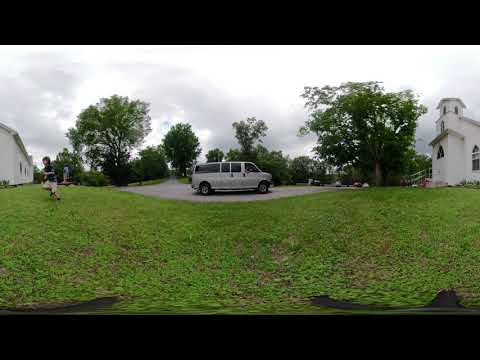The photograph features a silver minivan with chrome, five-spoke rims, prominently parked in the paved parking lot of an old, small, white church with a steeple. The van, oriented towards the right of the image, is equipped with two front doors and a sliding door behind the passenger side. Surrounding the parking lot are lush green trees, and the sky above is overcast with gray clouds.

To the left side of the photo, a little boy wearing a blue shirt and gray trousers runs across a grassy field. Behind him, a road stretches into the distance, flanked by another large tree. Further back, there is a white building that appears to be a house or perhaps part of the church complex, characterized by its stone exterior and arched windows.

The image has a black header and footer, giving it a letterbox appearance, making the picture itself longer than it is tall. On the right side of the photo, a large green tree stands adjacent to a white structure, potentially a house or a barn, adding to the quaint and serene atmosphere of the scene.